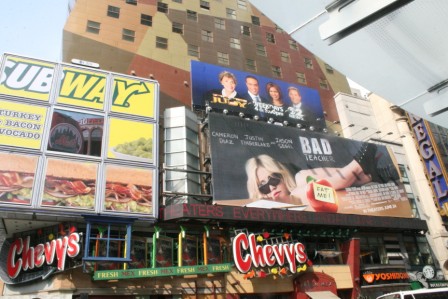The photograph is taken from beneath an awning of a building, shown in the upper right corner, adorned with white hanging lights. The image prominently features a multicolored building with several windows in the background, displaying distinct colored sections in orange, yellow, gray, and red hues. Beneath this building, a series of vibrant advertising signs catch the eye. 

On the right, there is a vertical, nine-section Subway advertisement promoting their Turkey Bacon Avocado sandwich, complete with images of the sandwich and avocado. Adjacent to this is a horizontal ad featuring a woman lying down, promoting the movie "Bad Teacher." Just above, another advertisement displays four individuals, likely promoting a television station as indicated by the number "22" on it.

Further below, the signs include a Chevy's logo and various other red and white advertisements. Another notable sign in this array reads "Yoshi" with additional undecipherable text. The layered and colorful assortment of ads and building façades creates a bustling cityscape image filled with commercial vibrancy.